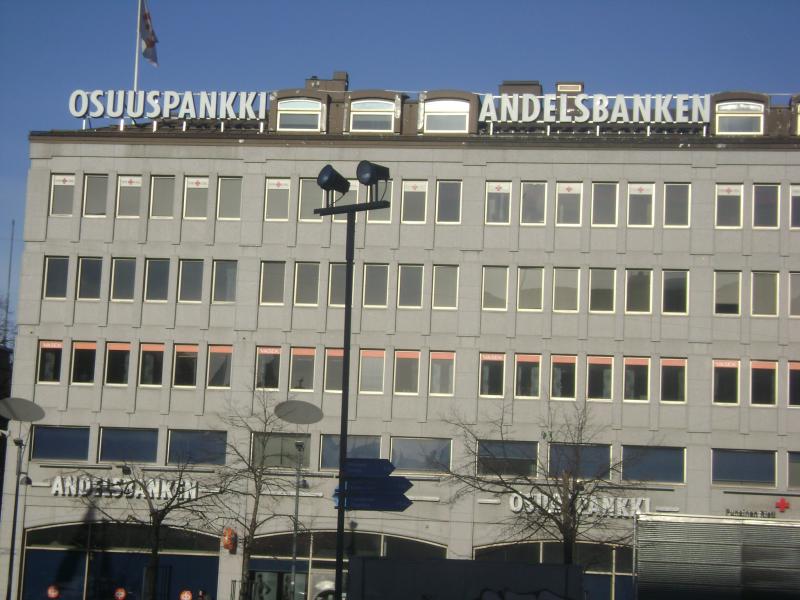This is a detailed outdoor daytime photograph of a large multi-story concrete building, likely situated in a city. The building features a symmetrical design with four main stories and a series of arches at the bottom level, which have horizontal rectangular windows underneath them. The upper three stories have rows of vertically oriented windows.

At the top left corner of the building, a flag is partially visible but obscured by shadows, making it difficult to identify its colors or logo. Prominently displayed at the top of the building is the text “OSUUSPANKKI” followed by “ANDELSBANKEN” in cutout letters affixed to the structure. The same text appears again in smaller letters above an arch on the first floor. 

In the lower right corner, there is a red cross sign indicative of a medical facility, although some texts are too fuzzy to decipher clearly. An orange clock or emblem is noticeable on one of the pillars. Additionally, a tall light post with two lights is positioned in front of the building, almost reaching the height of the structure itself. This architectural composition, coupled with the medical insignia, suggests that the building could potentially be a hospital or a bank with medical facilities.